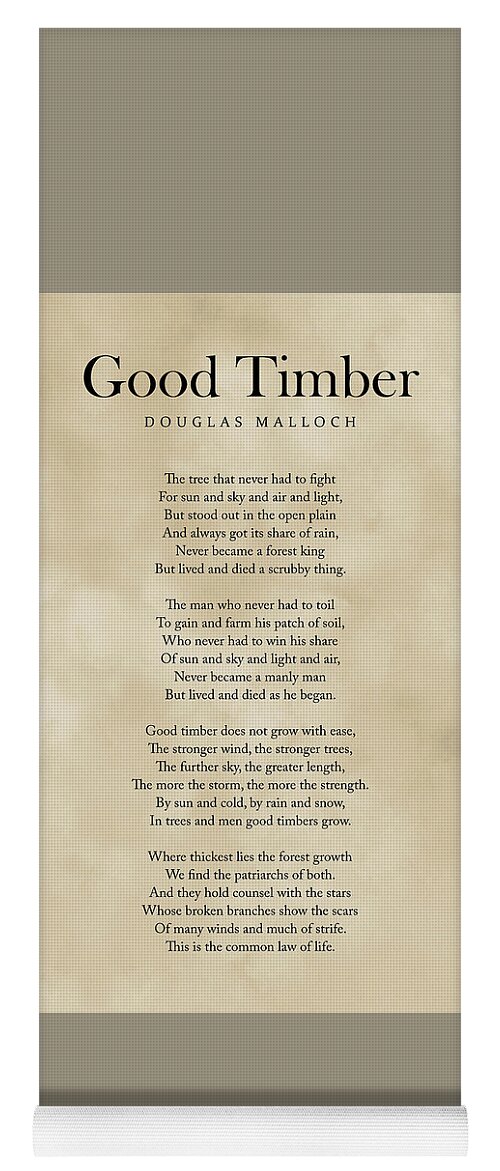The image showcases an elegantly designed poem titled "Good Timber" by Douglas Malloch. The poem is written in black font on a textured parchment background, with the title and author's name clearly distinguished—"Good Timber" in a larger font and "Douglas Malloch" in a smaller one. The text, structured into four detailed stanzas, is quite small and sits on a lighter brown section, contrasted by a darker brownish-gray perimeter at the top and bottom. The poem's visual presentation mimics an aged, old-fashioned style, possibly resembling a bookmark or a poetic stand. The background is a subtle blend of grayish brown, adding to the rustic and timeless aesthetic of the image.